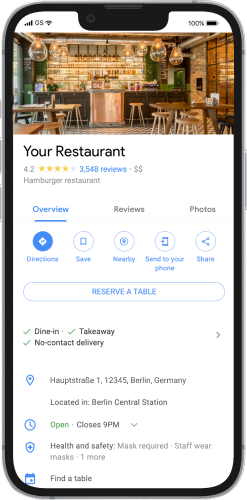In this detailed screenshot, we see what appears to be an image from an iPhone's display, distinctly outlined at the edges. The screen shows a Google Maps page showcasing "Your Restaurant," suggesting it may be a template or an example page. At the top of the page, there's a banner image depicting a bar area within a restaurant. Just below, the restaurant’s rating is prominently displayed: 4.2 stars from a total of 3,548 reviews. The establishment is categorized as a hamburger restaurant.

The interface features several tabs, with the "Overview" tab currently selected. Other available tabs include "Reviews" and "Photos." Below these tabs, there are various functional buttons labeled as "Directions," "Save," "Nearby," "Send to Your Phone," and "Share." Additionally, there’s a "Reserve a Table" button, enhancing user interaction options. The restaurant offers multiple service options, all marked with a tick: dine-in, takeaway, and no-contact delivery.

Further information reveals the restaurant's address, placing it in Berlin, Germany, specifically at Berlin Central Station. Curiously, there are placeholders showing numbers 1 through 5, reinforcing the suspicion that this may indeed be a template rather than a real listing.